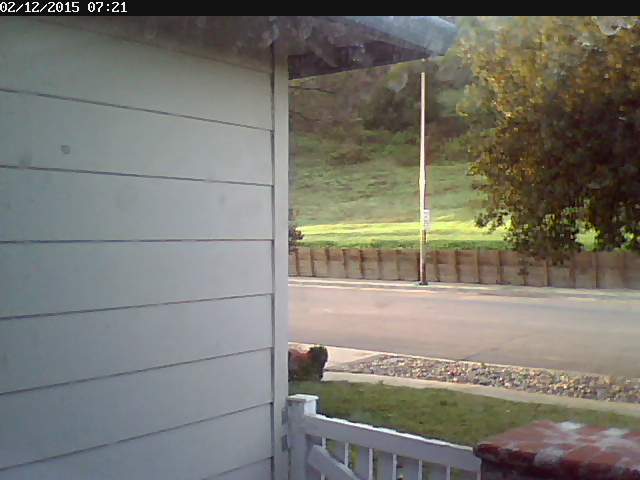This photograph, taken on February 12th, 2015 at 7:21 AM as indicated by the date stamp at the top, captures a serene, sunny day from the perspective of a patio. The patio appears to be part of a white-walled house. Part of a red stonework table is visible in the right corner of the image. In the foreground, there's a grassy yard extending to the edge of a gray road that runs horizontally through the middle of the image. On the opposite side of the street, a sturdy wooden fence marks the boundary of a large grassy field, with a sizable tree bearing green leaves standing prominently behind it. The tree’s branches extend partially over the sidewalk, casting subtle shadows. A black street pole is embedded in the concrete near the tree. A small brownish dog can be seen walking along the street. The capture exudes a peaceful, suburban morning ambiance.